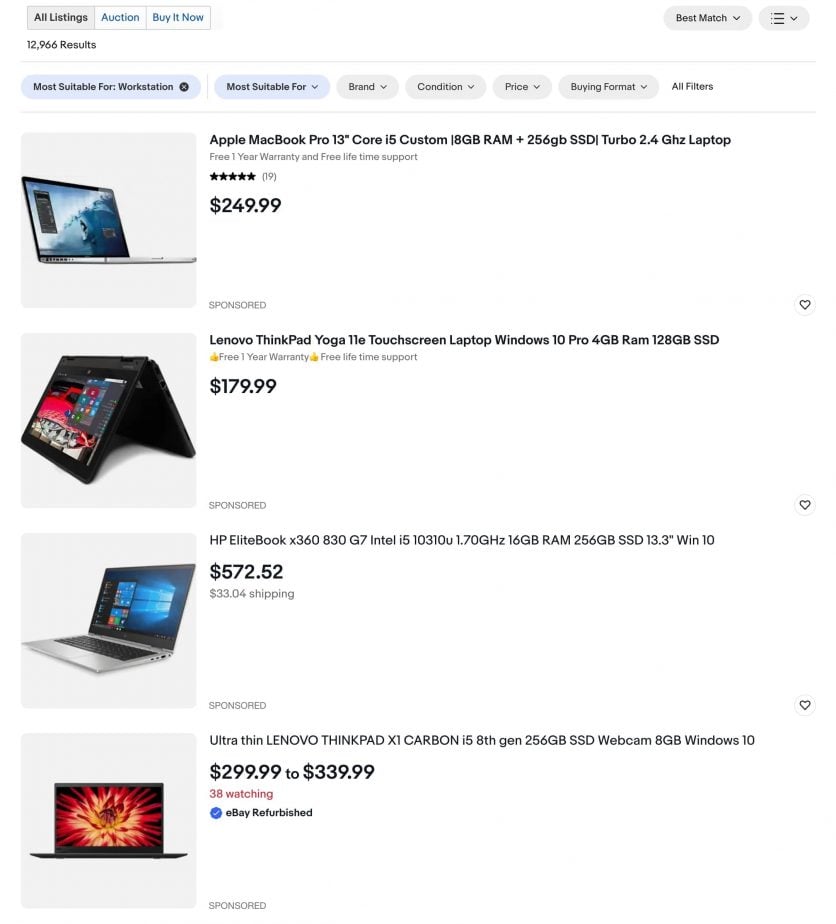The image resembles a typical eBay search results page, featuring listings for computers and laptops. There are approximately 12,966 results, with each listing marked as sponsored. The listings include a price tag and a heart icon in the corner for favoriting items. The upper right-hand corner displays sorting options such as "Best Match" and additional filters accessible via three horizontal lines. The visible laptop prices range from $179.99 to $572.52, with different shipping costs and buying formats, including auctions and buy-now options. The top of the page offers filters by workstation suitability, brand, condition, price, and buying format, allowing users to refine their search based on their preferences.